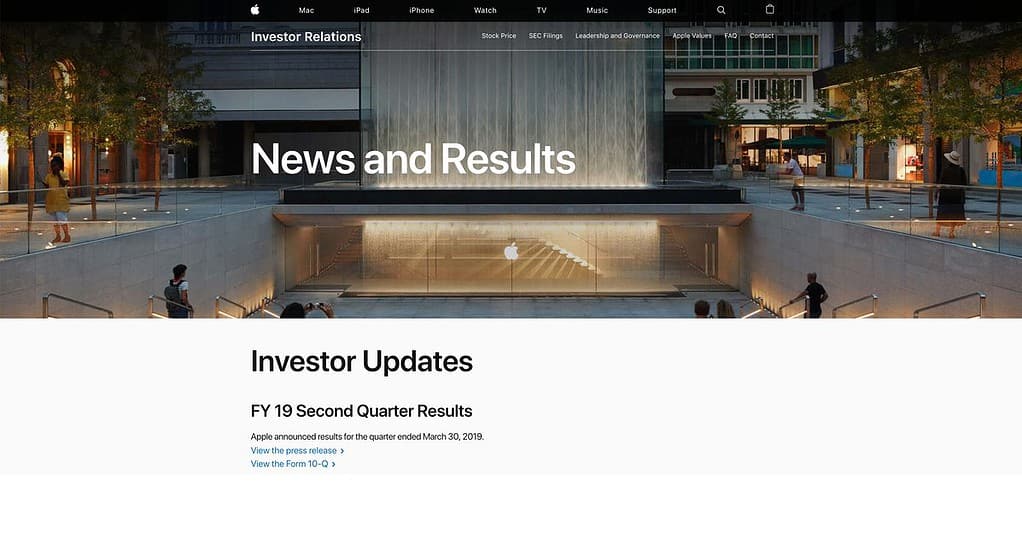An image showcasing the Apple Inc. Investor Relations webpage is displayed. At the top of the screen, a black navigation bar spans across, featuring a series of icons and labels starting from the left: the iconic Apple logo, followed by "Mac," "iPad," "iPhone," "Watch," "TV," "Support," and a search icon at the far right. Below the navigation bar, a prominent image shows an entryway with a set of steps leading up to sleek glass doors adorned with the Apple logo. A visually striking fountain cascades down like a waterfall in front of the doors.

Directly beneath the image, bold text reads "News and Results." Above this section, there are several tabs labelled "Investor Relations," "Stock Price," "SEC Filings," "Leadership and Governance," "Apple Values," "FAQ," and "Contact." Below the "News and Results" heading, specific details about investor updates are provided: "FY19 Second Quarter Results," followed by a brief summary indicating that Apple announced its results for the second quarter ending on March 30th, 2019. This section also includes two actionable links: one for the press release and another for the 10-Q form.